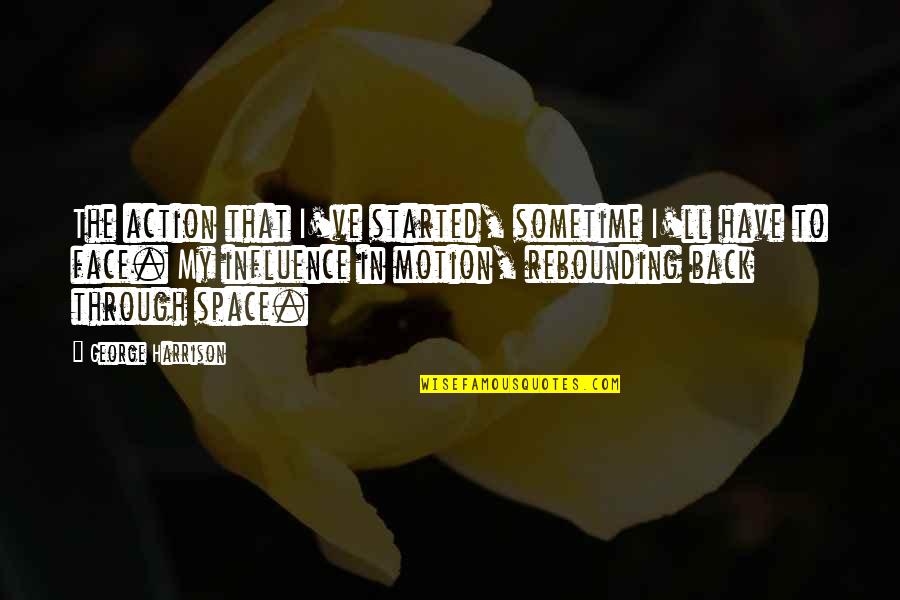This detailed rectangular poster features a quote from George Harrison, sourced from wisefamousquotes.com. The quote is printed in a bold black font against individual white rectangular backgrounds for each word, reading: "The action that I've started sometime I'll have to face my influence in motion rebounding back through space." The quote is broken into three lines – the first line includes "The action that I've started sometime I'll have to," the second line reads "face my influence in motion rebounding back," and the third line concludes with "through space," followed by "George Harrison." Below the quote, "wisefamousquotes.com" is displayed in yellow font.

The background of the poster is black, accentuating a central 3D shape that appears almost like a yellowish piece of popcorn or an abstract form with curving and folding segments, reminiscent of a roller coaster. There may be an illusion of a hand with bent fingers in the backdrop, contributing to the texture and depth of the image.